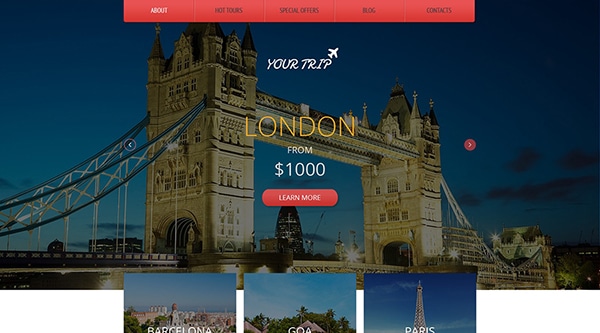The photograph is a striking nighttime image showcasing the iconic Tower Bridge in London, England. This majestic bridge, notable for its twin towers designed in a late Victorian Gothic style, features a suspension span supported by large cables that anchor to the ground, allowing for vehicular traffic to pass through archways at the base of the towers. High above, the two towers are connected by a horizontal walkway, approximately four stories up, giving the appearance of castle turrets crowning each tower. The sky is tinged with the hues of either dusk or dawn, with gray clouds forming a dramatic backdrop.

Across the center of the image, large yellow text states "London" and an enticing offer "from $1,000" in white. Beneath this, a prominent red button labeled "Learn More" in white letters directs potential travelers for additional information. Just below this call-to-action, three smaller images are partially visible, suggesting travel destinations such as Barcelona, with its distinctive skyline; a locale featuring pyramids, possibly Giza; and Paris, dominated by the silhouette of the Eiffel Tower. A vivid red header crowns the top of the display, adding to the overall vibrancy of this enticing travel advertisement.